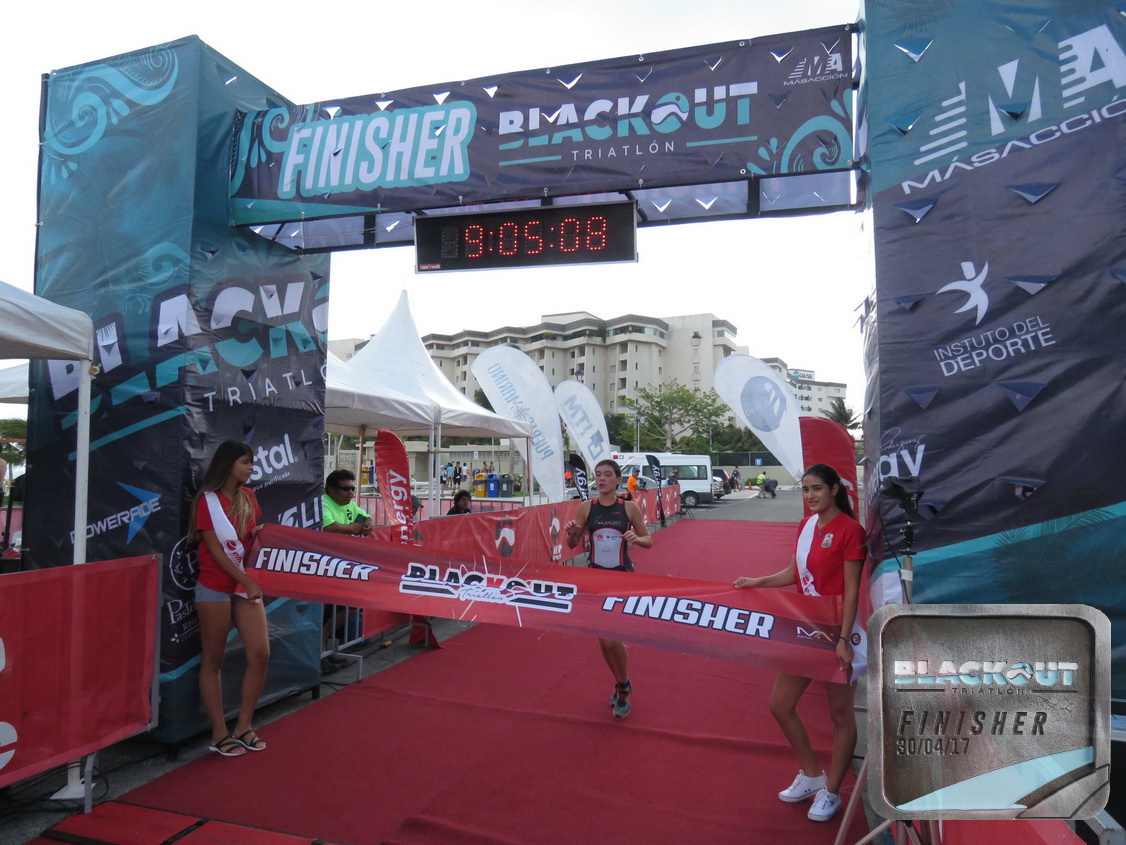At the finish line of the Blackout Triathlon, a meticulously arranged scene unfolds. A vinyl archway, supported by scaffolding and adorned with a printed multicolored blue and black design, prominently displays "Blackout Triathlon Finisher" and a timer reading 9:05:08. Below this, two young women in red t-shirts and short shorts hold a red banner emblazoned with "Finisher," ready for a participant to cross. The runner, clad in a spandex tank top, appears exhausted but determined as they approach the ribbon, likely achieving first place. Surrounding the finish line is a vibrant red-carpeted area filled with spectators, barricades, and signs, set against the backdrop of urban apartment buildings or a hotel and van. The scene is completed by a small stage decorated in teal, black, blue, and white with additional signs, some in Spanish, celebrating the event held on April 30th, 2017. This meticulously organized finish line captures the culmination of the athlete’s grueling nine-hour endeavor.